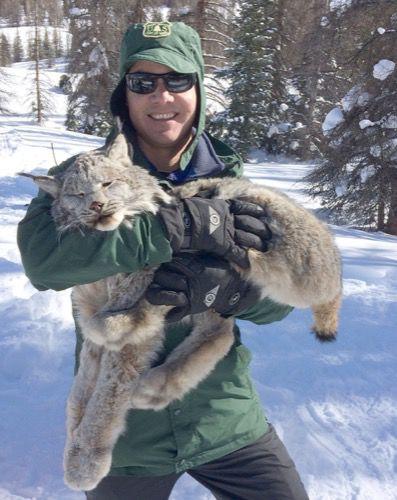In this vertically oriented photograph, a snowy winter scene frames a man dressed in a green jacket adorned with a badge and text on his hood, indicating he might be a park ranger or wildlife official. He is also wearing gray pants or possibly black snow pants, thick black gloves, and black sunglasses. On his head, he sports a green cap with an emblem. He stands amidst a backdrop of snow-covered pine trees, suggesting a deep winter setting, possibly in a forest or even a ski resort area.

The man holds a large, wild feline creature in his arms, which appears to be a bobcat. The cat's fur is a mix of beige, whitish, grayish, and slightly creamy colors, conveying a lush and furry appearance. The cat's eyes are closed, and although its legs are not limp, suggesting it might be sleeping, there is also a possibility it could be deceased, as indicated by blood on its face. Both the man and the cat face the camera, with the man smiling broadly despite the cold and harsh winter environment surrounding them.